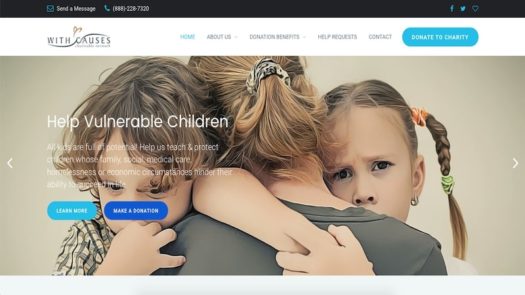A detailed web page screenshot is captured, predominantly showcasing a black banner at the top with an invitation to "Send a Message." This banner features a blue email envelope icon and a blue handset icon followed by a phone number: 888-226-7200. To the right of this black banner, social media icons for Facebook, Twitter, and a heart symbol are displayed.

Below, a white banner contains the word "Causes," accentuated by an upward sweeping graphic and a gold heart. The site's navigation menu includes a blue-highlighted "Home" button with additional options: "About Us," "Donation Benefits," "Help Request," "Contact," and another blue button labeled "Donate to Charity."

Dominating the main area of the web page is an emotional image of a little girl with two braids in her hair, accompanied by a woman and a young boy who appear to be embracing each other, all facing the camera. Overlaying this touching image, white text reads "Help Vulnerable Children." The image also includes two prominent blue buttons: one saying "Learn More" and the other "Make a Donation."